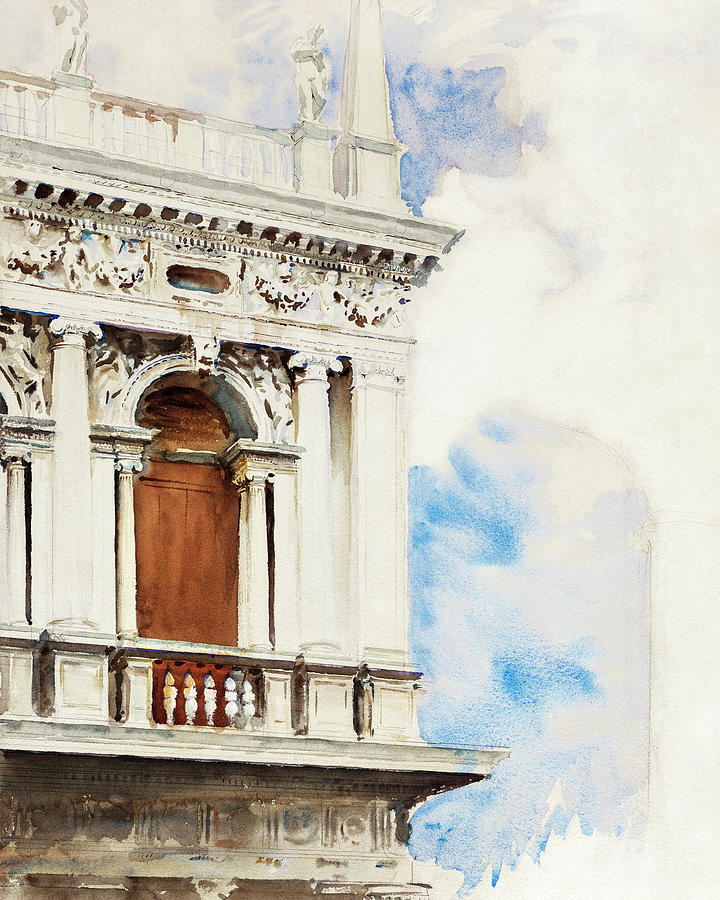This is a detailed watercolor painting of an architectural building, showcasing a historical structure. On the left side of the image, you can see the corner of an old building with intricate masonry work and white columns that support the upper level. Particularly detailed on the left, the painting features a prominent brown arched doorway, suggesting an entrance to an upper room. Above the doorway is a balcony with a light brown railing, which appears to provide a space to stand although no individuals are depicted.

The structure boasts impressive carvings above the doorway and on the stanchions. An overhang with ornate carvings extends above the balcony, adding to the building's aged and historical appeal. Higher up, there is a roof with a trapezoidal feature that resembles a gutter. Additionally, the rooftop hosts several short statues of men, accompanied by a decorative guardrail, potentially for both safety and ornamentation. To the right of the building, the sky is a serene blue partially obscured by white clouds, covering about two-thirds of the sky.